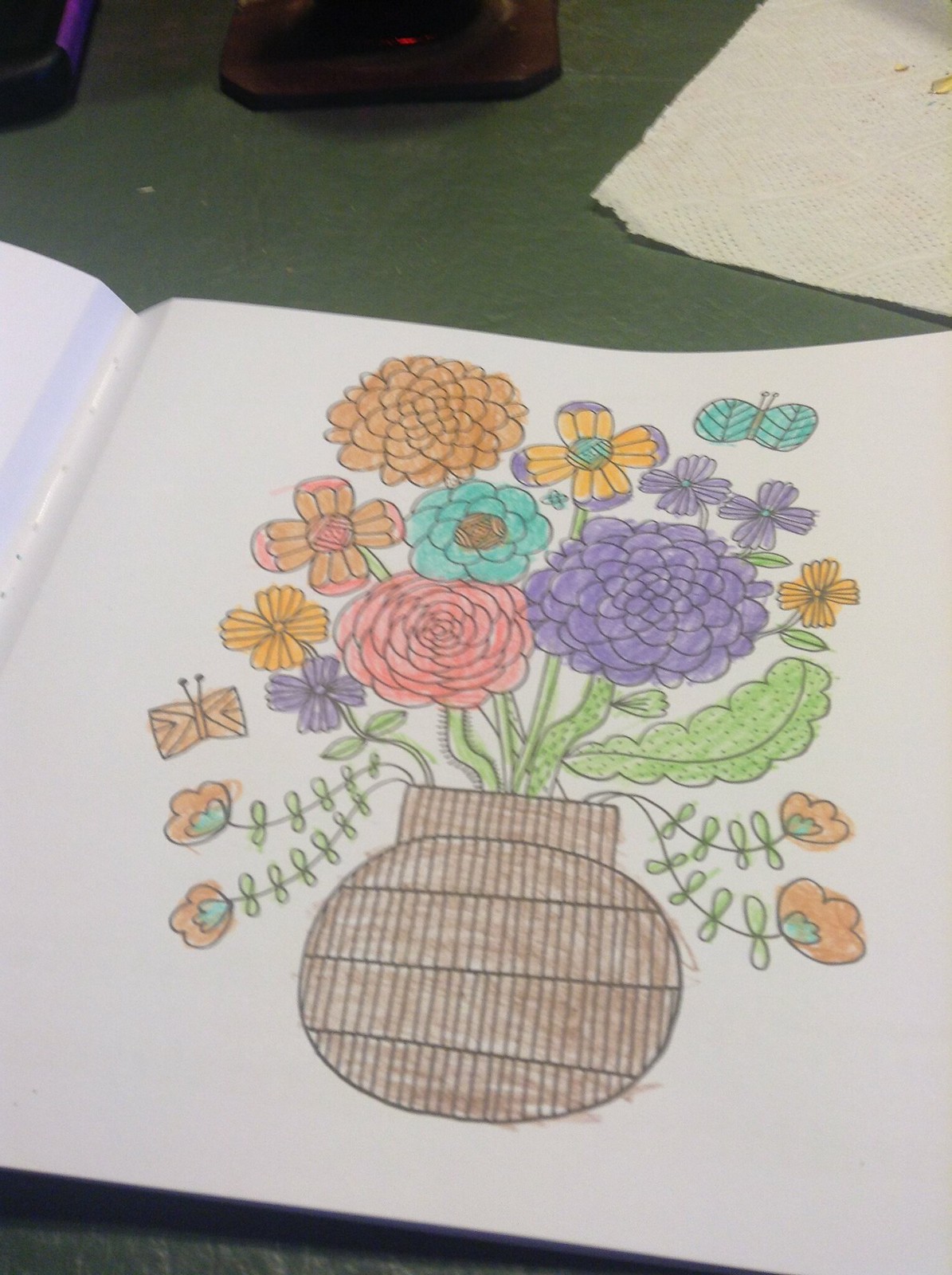A black marker sketch on a white sheet of paper depicts a vase created from a simple circle, adorned with three horizontal lines and an opening at the top resembling a chimney. This vase features vertical brown stripes and additional brown squiggly lines that form an intricate pattern. Emerging from the vase is an array of flowers in vibrant shades of orange, purple, aqua, and pink, alongside green leaves and stems. Two butterflies, colored in aqua and orange, hover delicately around the floral display, adding an extra touch of life and color to the composition.